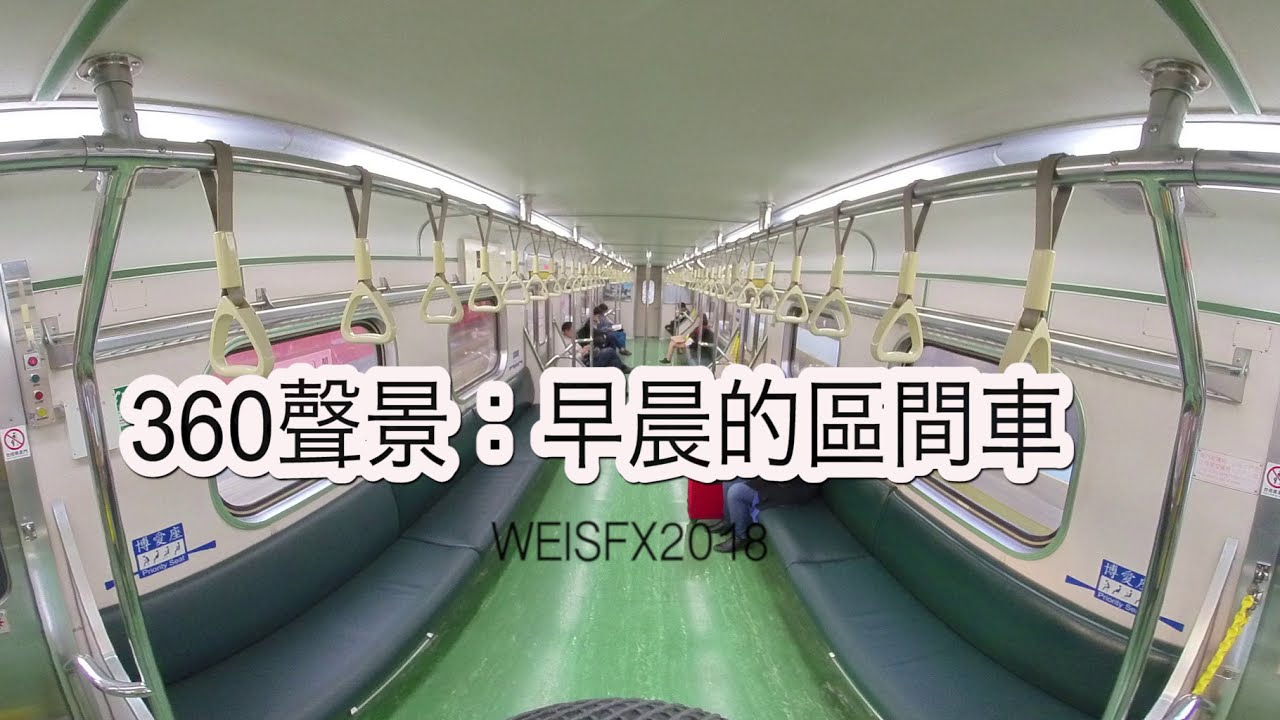This is an interior photograph of a train or subway car. The walls and ceiling are white, giving it a clean and bright appearance. A shiny metal bar runs parallel to the ceiling, adorned with gray looped straps and white triangular handles spaced evenly every two feet. Thin fluorescent lights extend across the length of the car near the ceiling edges. The floor is light green with blue edges. There are blue seats along both sides of the train, and at the far back, a few people are seated, making the car appear lightly populated with around four passengers.

Prominently featured in the foreground is black writing on a white background that reads "360" followed by six Chinese characters, heavily outlined in white. Below this, in smaller black letters, it says "WEISFX 2018." Behind this text, on the right side of the car, there appears to be a person in a wheelchair positioned near the blue bench seating. The overall impression is of a well-lit, spacious, and relatively empty train car, designed for accessibility and passenger comfort.